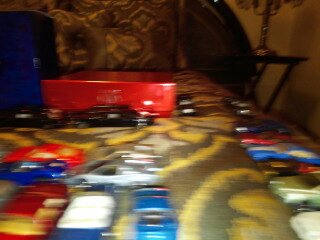The image depicts a living room featuring a brown and gold couch with intricate golden designs, partially visible due to the blurriness. Scattered across the couch and carpet are numerous Hot Wheels cars in various colors including red, blue, white, and black. On the left side, cars are arranged vertically, while in the right corner they are lined up horizontally. Toward the back, a red box lies flat with a blue box standing beside it, and a car positioned adjacent to the red box along with two more cars in front of these boxes. In the background, a black table supports a lamp, accompanied by a black wooden piece. The photograph's overall scene suggests a child with an evident passion for toy cars, as they are spread across the room in a playful disarray.